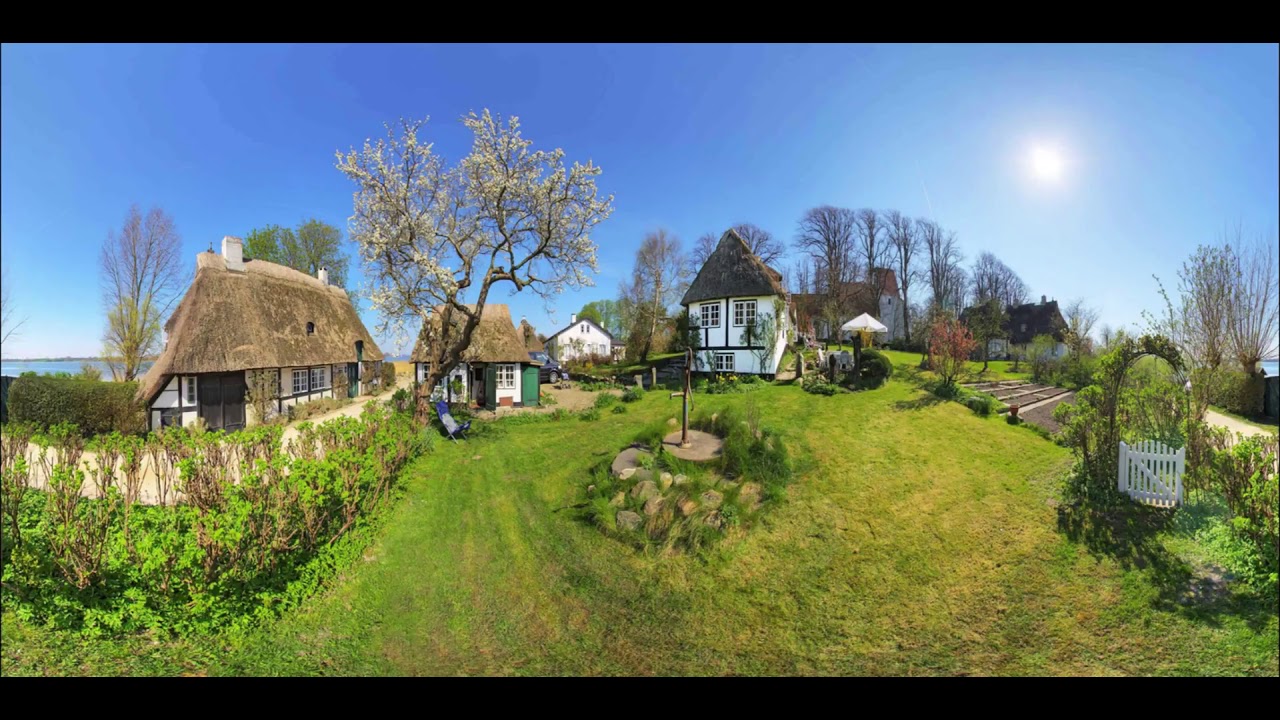This 360-degree panoramic image, possibly captured from a drone, showcases an idyllic cluster of quaint European-style beachside cottages nestled in a lush, grassy area. The cottages, with their white stucco walls and steep, possibly straw-like shingled roofs, exude an aura of historic charm akin to structures that might be centuries old, reminiscent of a Norwegian seaside. The scene features a dirt driveway meandering up to the cottages, flanked by manicured shrubs and a white picket fence leading into a probable garden. Central to the image is a rocky area featuring a cement circle and a water pump, suggesting a well. Among the cottages, one is distinguished by garage doors to its left and a main entrance on the far right, while another smaller guest house cottage sits nearby. Additionally, a two-story cottage perches slightly uphill. Encompassing the cottages are beautifully flowering trees, vibrant bushes, and an array of lush vines, all under a brilliantly clear, cloudless blue sky with a hint of water visible on the distant horizon. The pristine and almost surreal quality of the landscape hints at the possibility of a computer-generated image, enhancing its enchanting and inviting atmosphere.